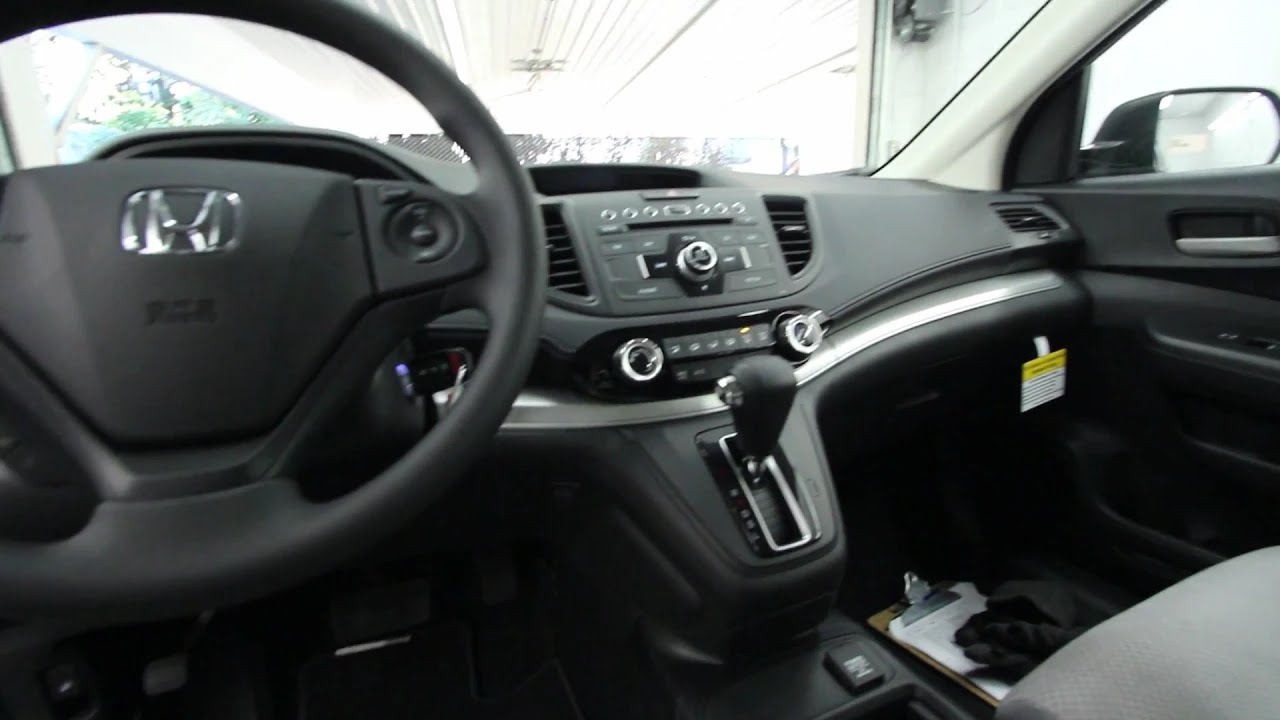This image captures the detailed interior of a modern Hyundai, identifiable by the logo on the steering wheel. The perspective is from the driver's seat, showcasing a sleek black interior enhanced with some silver or chrome trim pieces. The clean and well-maintained dashboard features prominently in the center of the image, displaying a gear shift integrated with the dashboard, radio, and air conditioning vents and controls. The center console is a focal point, along with the visible steering wheel on the left side. In the passenger seat footwell, a clipboard with papers and a pair of gloves is noticeable, suggesting some recent activity related to note-taking. The vehicle is stationary, likely parked inside a spacious building. Outside the windshield, an overhead structure resembling a roof or awning partially obstructs the view, with glimpses of trees and sky visible beyond, while the passenger’s side window provides a glimpse of a nearby white wall. The overall impression is of a new or well-kept model with advanced features, highlighting a visually appealing and functional interior.